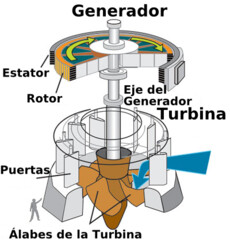The image is a detailed diagram of a large-scale turbine generator, labeled in Spanish. At the top of the diagram is a component labeled "Generador" (Generator), followed by vertical sections labeled "Estator" (Stator) and "Rotor" (Rotor). A central vertical post, or "Eje del Generador" (Generator Shaft), runs down the middle. The bottom section features another cylindrical component marked "Turbina" (Turbine), with additional labels "Puertas" (Doors) and "Alabes de la Turbina" (Turbine Blades). The scale of the contraption is emphasized by a small likeness of a person in the bottom left corner, indicating the massive size of the facility. The diagram also includes arrows indicating the direction of rotation for the turbine.